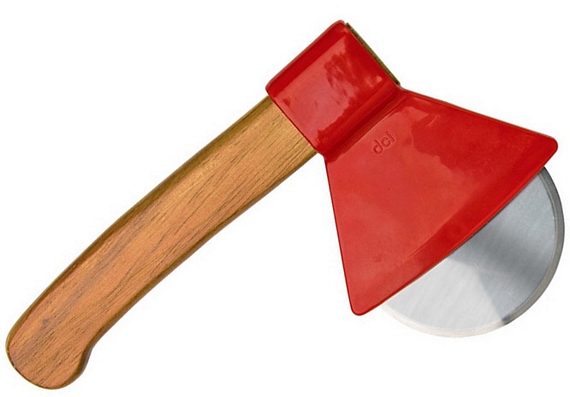This image features a unique, novelty pizza cutter designed to resemble a traditional axe. The cutter has a glossy, medium brown handle that mimics the look of wood, typically seen on tools like hammers or axes. The handle extends to a red, triangular housing made of glossy material that appears plastic-like, and this housing encases the circular, shiny silver blade. The blade is reminiscent of those used in standard pizza cutters, designed to slice through pizza efficiently. The entire object rests against a plain white background, offering no additional context clues.